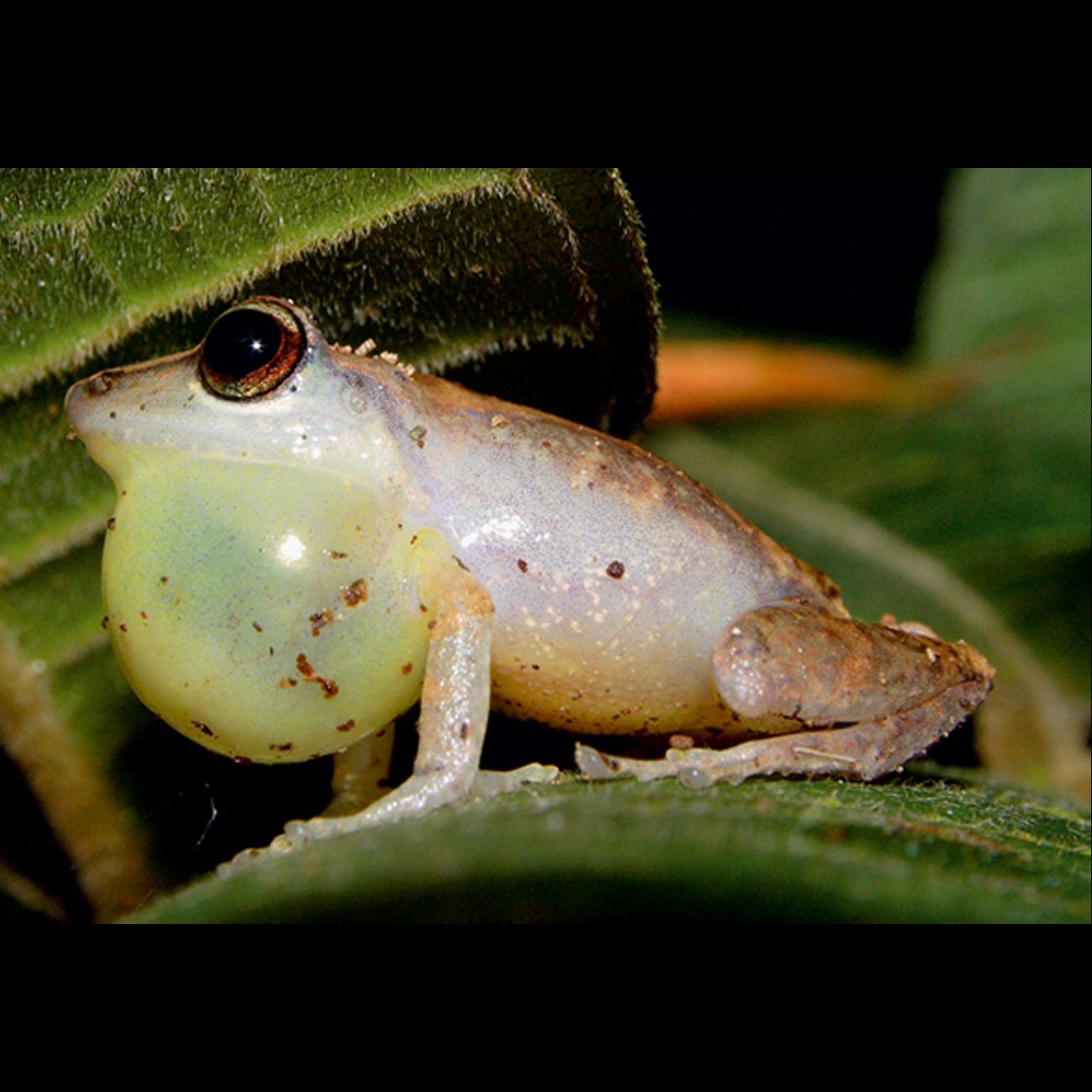The image features a small, brown and white frog perched on a dark green leaf. The leaf looks somewhat furry and provides a contrasting backdrop for the frog. Its throat is highly inflated, forming a yellowish, translucent balloon-like structure, suggesting that it might be in the process of croaking or consuming something. The frog's large, brown and black eyes, with their circular black pupils, add to its striking appearance. The scene is set outdoors, possibly at night, indicated by the darker, blurry background, hinting at a wildlife setting. The picture is framed with black rectangles at the top and bottom, adding a distinctive visual border to the composition.